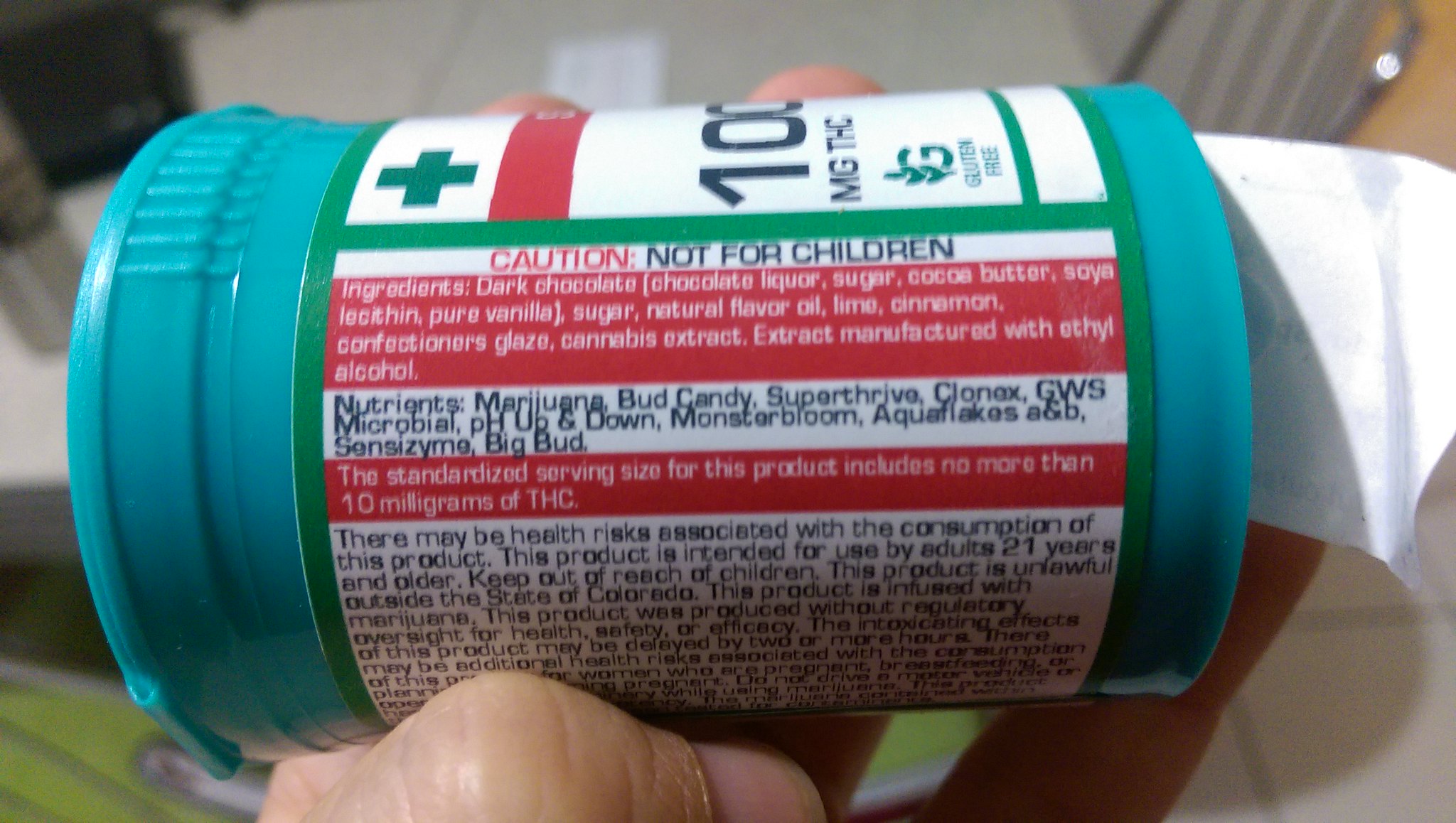The image depicts a close-up of a turquoise bottle, which appears to be a form of marijuana or cannabis-infused candy. The bottle, held sideways, features a detailed label designed with green, white, and red elements. Prominently displayed in red text is a cautionary note indicating the product is "not for children." The visible portion of the label includes the text "100 MG THC," suggesting the bottle contains 100 milligrams of THC, the active ingredient in cannabis.

The label highlights the product's ingredients, listing dark chocolate, sugar, natural flavor oil, lime, cinnamon, confectioners glaze, and cannabis extract, which is manufactured with ethanol alcohol. The standard serving size is specified as no more than 10 milligrams of THC. Additionally, the label includes an extensive warning section emphasizing that the product is intended for adults aged 21 and over and should be kept out of the reach of children.

In the image, a thumb holding the bottle can be seen at the bottom, and the blurred gray background includes a black object in the top left corner. A partial white receipt is visible on the right-hand side, further emphasizing the context of the product as a consumer item.